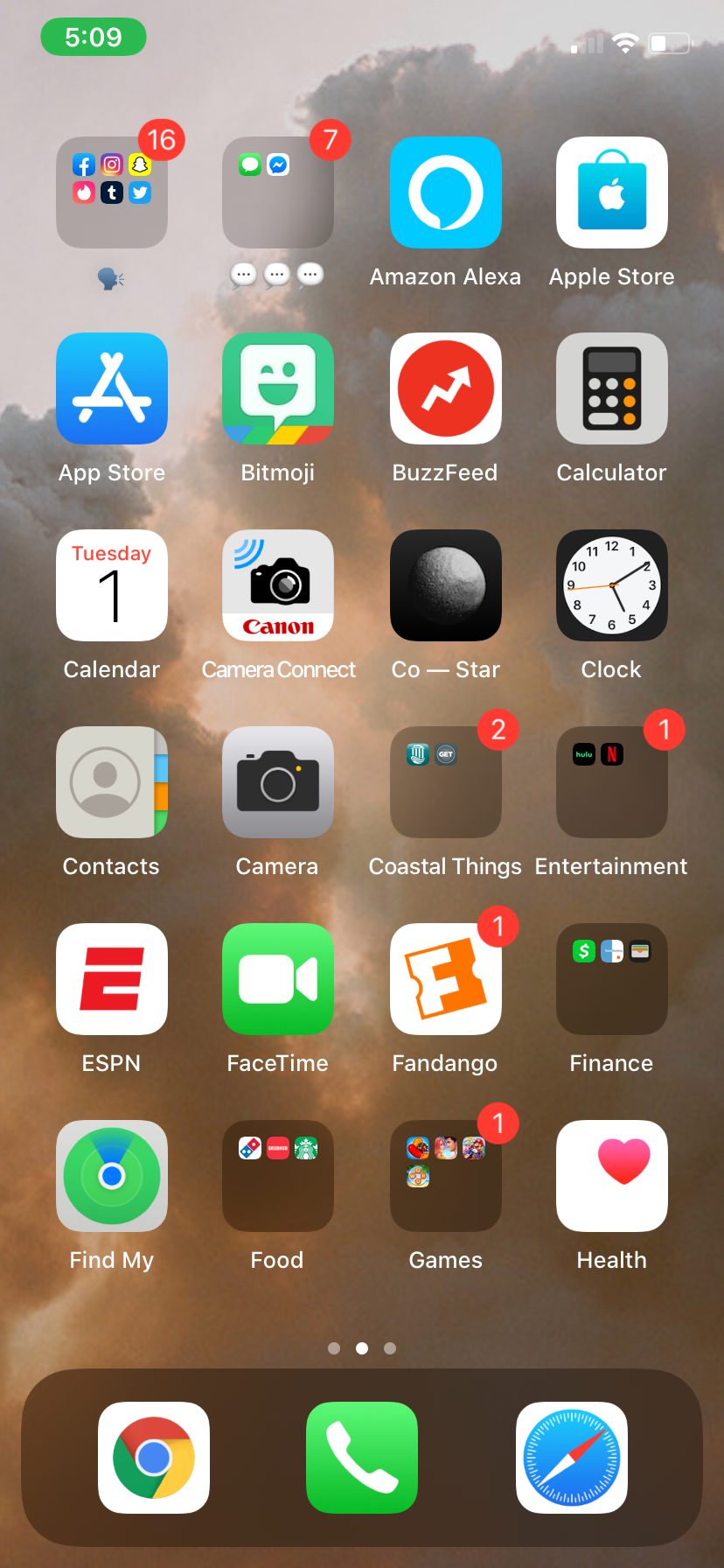Screenshot of a smartphone home screen taken at 5:09 PM, showcasing a sky with dark gray clouds as the background. Icons are neatly organized into folders. One gray folder contains various utility apps including 'Amazon Alexa,' 'Apple Store,' 'App Store,' 'Bitmoji,' 'BuzzFeed,' 'Calculator,' 'Calendar,' 'Camera,' 'Kinect,' 'Kodash,' 'Star,' 'Clock,' 'Contacts,' and a second instance of the 'Camera' app. This folder displays a notification with the number 16 in white on a red circle.

Another gray folder with two icons labeled 'Chat' and 'Messenger' shows a notification with the number 7. Other folders visible include 'Entertainment' (with apps like ESPN, FaceTime, Fandango, marked with the number 1), 'Finance' with three icons, 'Find My' marked with the number 1, 'Food' with three icons, 'Games' with four icons labeled with the number 1, and 'Health.'

At the very bottom of the screen, three primary app icons are shown: Google Chrome, the phone dialer, and Safari.